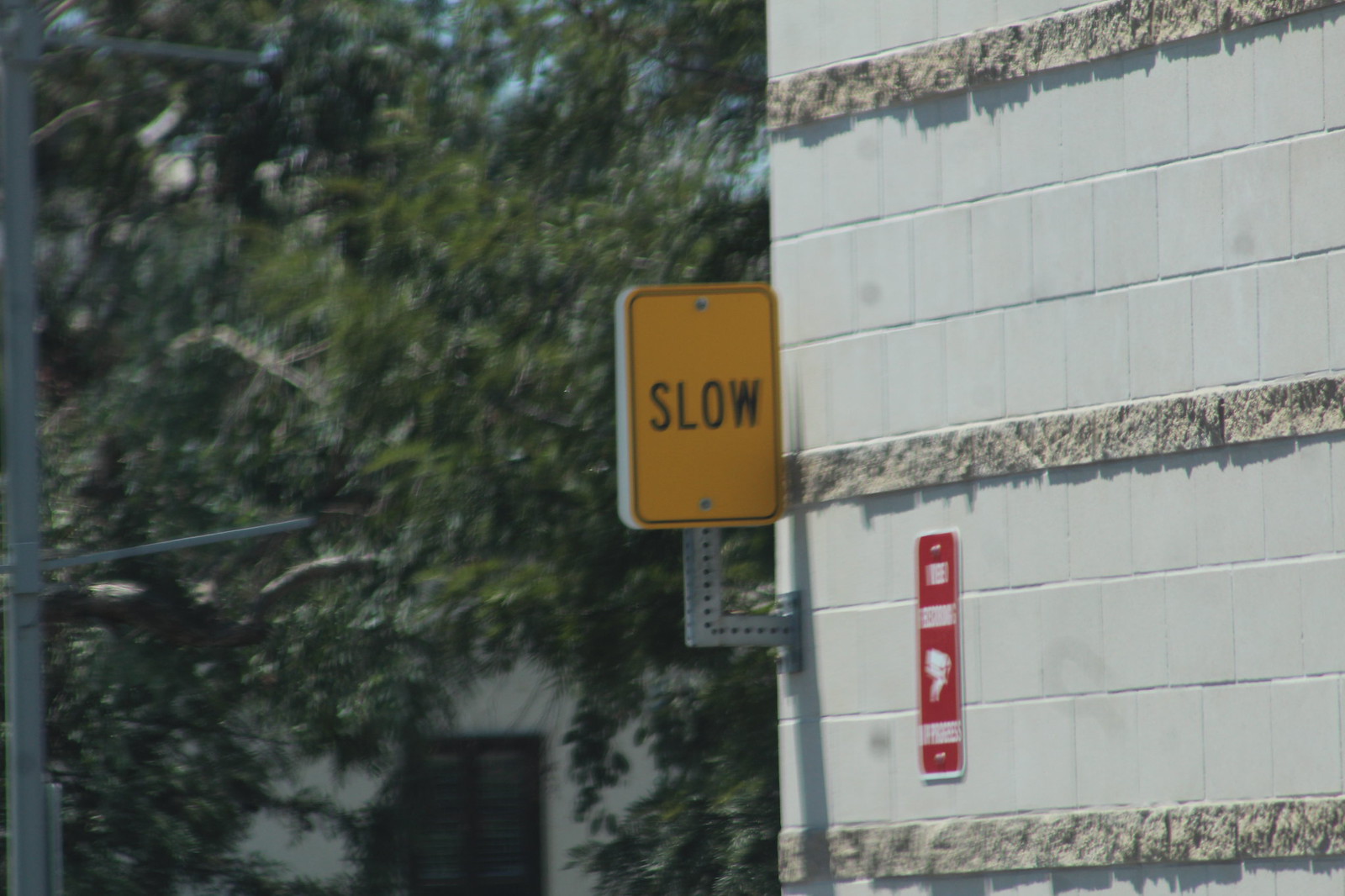The photograph depicts a white brick wall of a building, interspersed with stones embedded between the bricks, giving it a textured appearance. On the side of the wall, there is a prominent red sign, and protruding from the wall is a yellow sign with an L-shaped handle bearing the word "SLOW." The image, slightly blurred and lacking sharp focus, suggests it was taken from a moving vehicle. In the background, dark green trees partially obscure a white house with dark brown doors, adding depth and context to the scene.